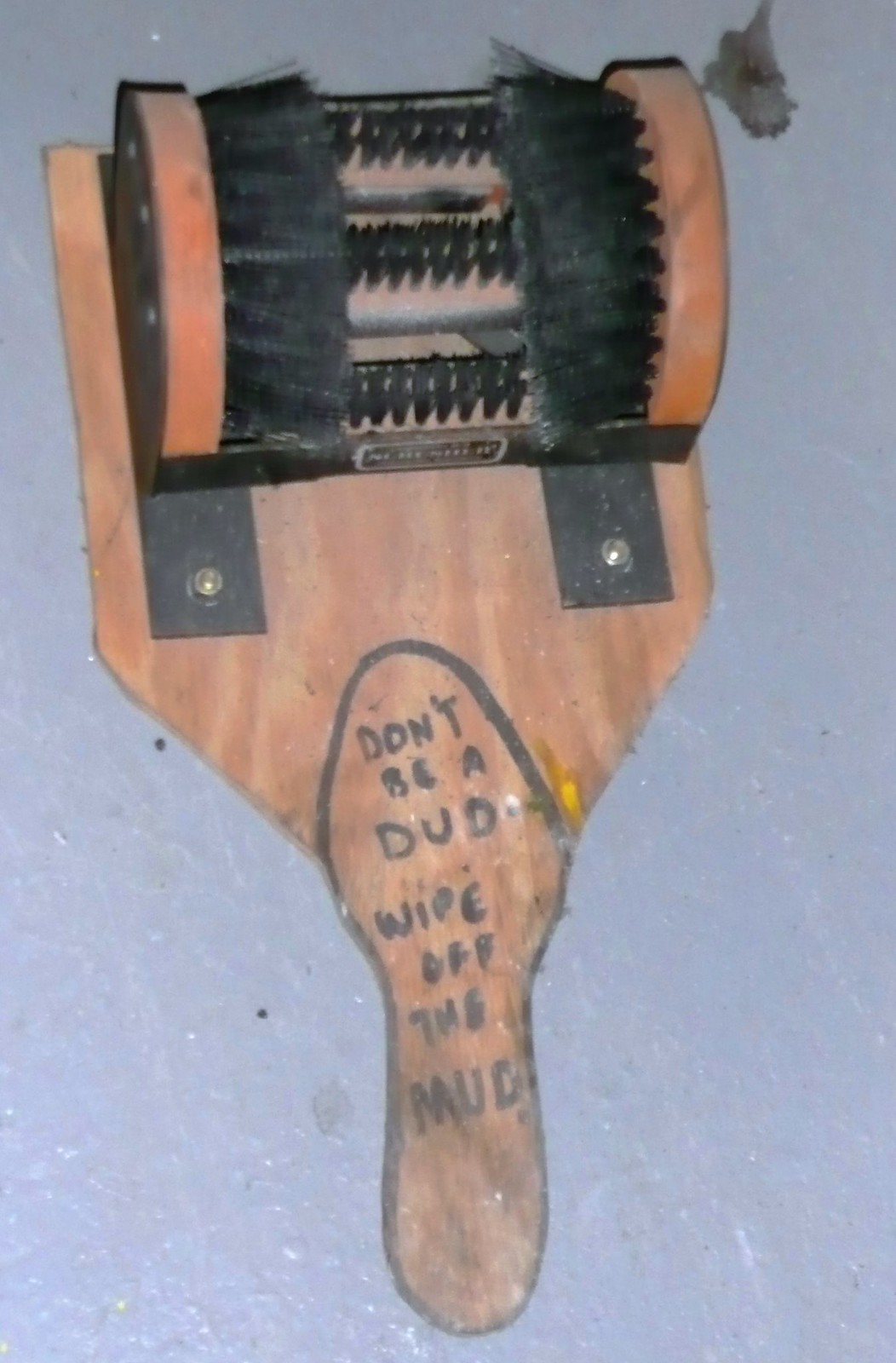The image depicts a boot scraper designed to remove mud or dirt from shoes. The device is placed on a solid, textured white surface that appears to be slightly uneven and reflective, suggesting it has been painted. The boot scraper itself resembles a paddle, with a square top curving into a rounded handle. It is constructed from wood and is bolted to the surface, with visible bolts near the top. The wooden base features an outline of a foot at its start, emphasized with black outlines and accompanied by the inscribed words "DON'T BE A DUD, WIPE OFF THE MUD" in capital letters.

Mounted on the base with metal brackets is a metal contraption hosting an array of black-bristled brushes: two large, round brushes facing inward to clean the sides of shoes, and three upward-facing brushes for cleaning the soles. Additionally, there is a gray handle in the top right corner of the device, contributing a shadow to the textured, white surface beneath it.